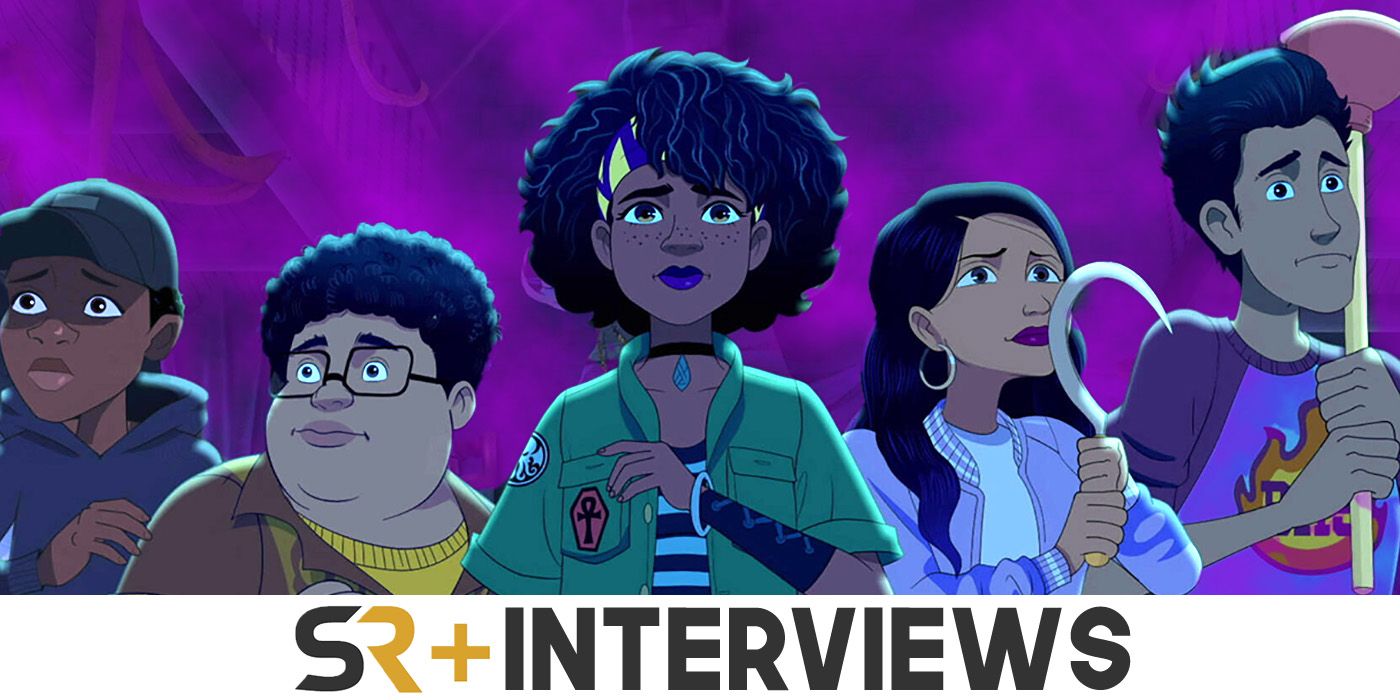The promotional image for an animation displays five teenagers of African-American descent against a vibrant background of various blue hues mixed with dark pinks. At the bottom of the image, the text "SR plus interviews" is displayed, with the 'S' and 'interviews' in black font, while the 'R' and 'plus' are in a goldish orange color. In the center stands a young woman with short full curly hair, wearing a green military-style coat adorned with Egyptian symbols, a black and white striped shirt, a yellow and blue striped bandana, blue lipstick, a choker necklace, a bracelet, and a fabric cuff on her left forearm. To her left is a shorter woman with a bit of an afro and glasses, dressed in a yellow t-shirt under a brown jacket, and a boy in a green ball cap and a blue hoodie, appearing frightened with his hand on the shoulder of the person next to him. To the right of the central figure is another young woman with long black hair, big gold hoop earrings, a white t-shirt under a purple jacket, holding a scythe. She looks concerned with dark red lips. Behind her, a tall young man with wavy and thick short hair, wearing a two-tone blue shirt with a flame logo, clutches a toilet plunger in a defensive posture. The characters convey a mix of emotions ranging from resolute to worried and frightened, adding a dynamic and intriguing element to the image.